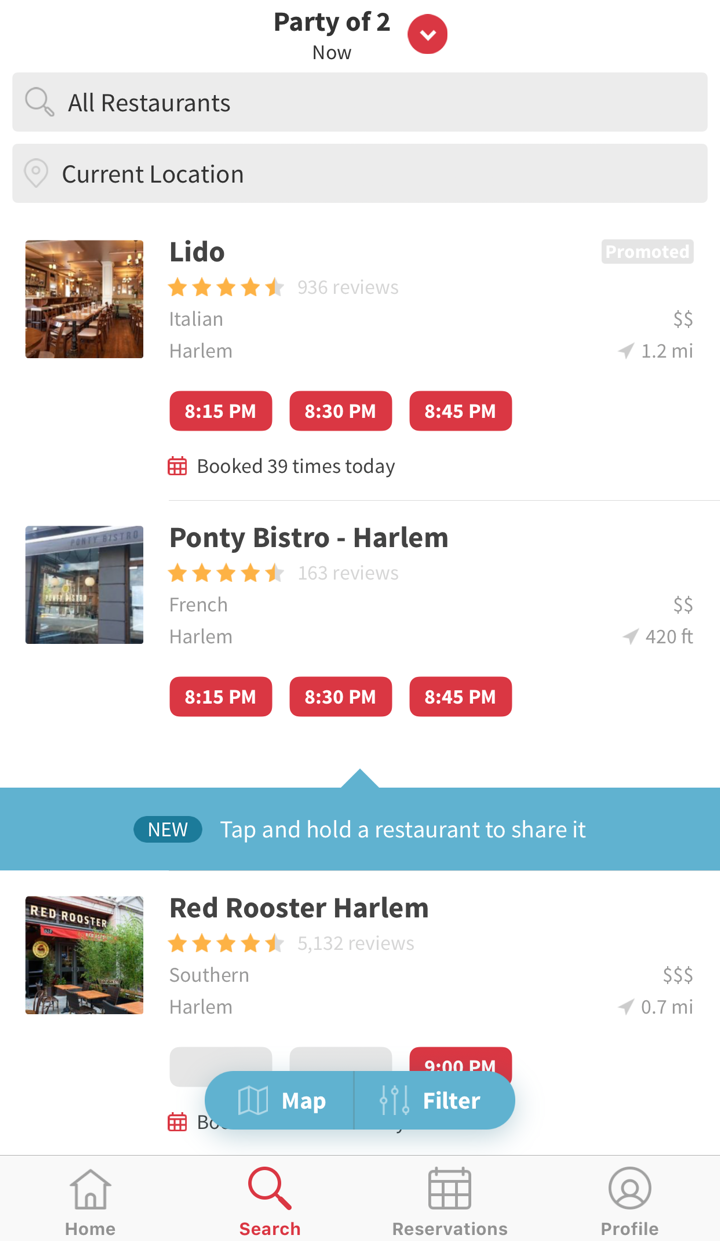The image appears to be a screenshot of a mobile app, likely Yelp, given the red and white color scheme. The screen displays the "Search" section, indicating that the user is looking for restaurants. At the bottom of the screen, there are navigation options labeled as Home, Search, Reservations, and Profile. The current search results are for Italian and Southern cuisine restaurants located in Harlem.

Three specific listings are visible:
1. **Lido**: This Italian restaurant has a rating of 4.5 stars and is located 1.2 miles away. 
2. **Ponty Bistro**: A French restaurant situated 420 feet from the user, offering booking times starting at 8:15 PM.
3. **Red Rooster**: Known for its Southern and soul food, this restaurant is 0.7 miles away with reservation times available from 9 PM. It is also noted as the most expensive option among the three.

The app includes options to book tables, indicating available reservation times, which implies that the user was searching for dinner options later in the evening.